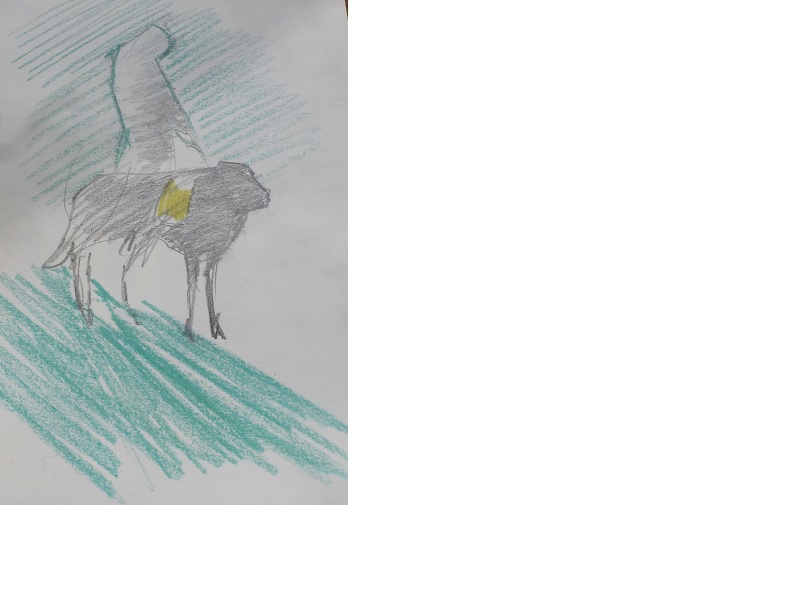This image is a detailed color drawing on a plain white piece of A4 sketch paper, captured in a photograph. It appears to be created primarily with crayons and a regular pencil. The drawing features an ambiguous animal, either a dog or cow, facing the right side of the image, depicted in a rough, black silhouette. The animal has an uneven number of legs, including two visible front legs, one skinny rear leg, and one larger leg, along with a visible tail but no eyes. 

A distinct yellow scarf is wrapped around the animal's neck, likely indicating it is a dog. Behind this animal stands the silhouette of a person, seemingly pointing toward the ground. The bottom of the image is filled with diagonal scribbles of green crayon, representing patches of grass, drawn in a haphazard manner both from the upper left to the lower right and from the upper right to the lower left. The green scribbles do not cover the entire bottom portion but appear as rough patches, creating a simplistic, textured background.